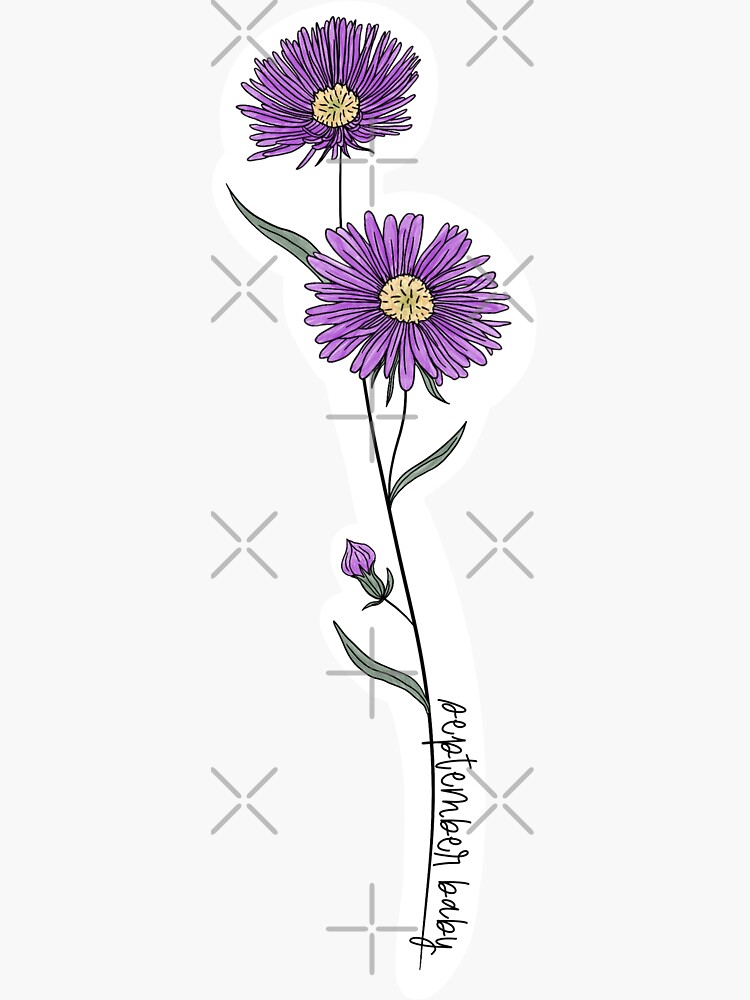The image is a drawing, likely digital, of three purple flowers with a distinct white outline on a predominantly white background. The main focus features two fully bloomed flowers with yellow centers standing prominently near the top, while a smaller, unopened flower bud is positioned near the base of a skinny green stem that extends vertically from the bottom to the top of the image. The stem is adorned with three green leaves at various points. Surrounding the flowers are watermark-like symbols—gray X's with circles at their intersections, resembling sparkles or glitter. Along the stem, the words "September baby" are delicately written in cursive, aligning vertically with the stem's edge.